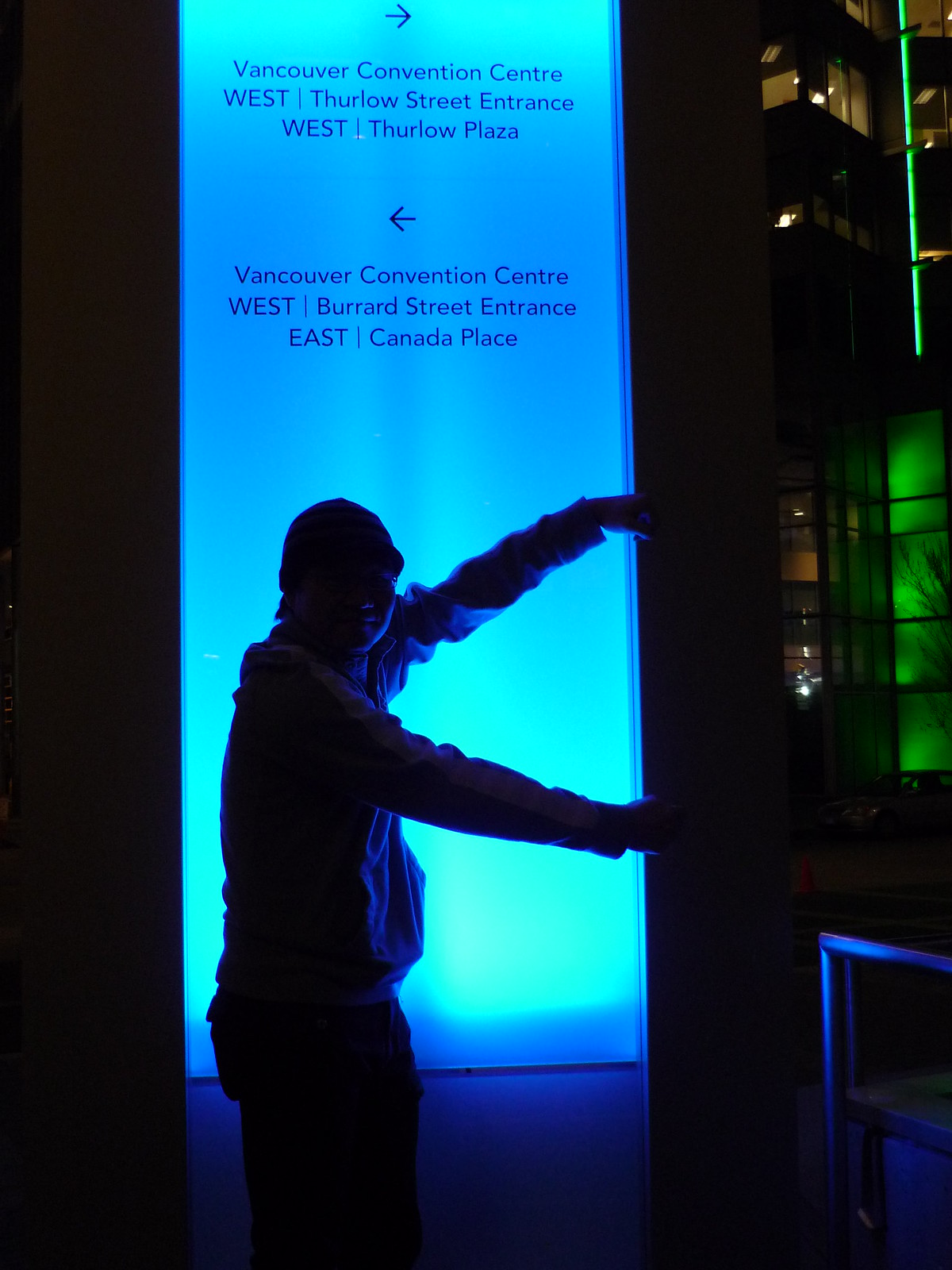This is a nighttime color photograph featuring a solitary individual standing in front of a brightly illuminated, rectangular neon sign. The scene is mostly dark, emphasizing the vibrant neon sign that serves as the focal point. The individual, likely a man wearing a beanie hat, long-sleeved shirt, and dark pants, is seen from behind and slightly sideways, with arms stretched out in a V shape as if interacting with or holding the sign. Despite the dark surroundings, the neon sign vividly lights up in varying shades of deep ocean blue with lighter blue hues towards the center. 

The sign serves as a directional guide in Vancouver, with black or bluish-black text and arrows indicating various locations. An arrow to the right points towards the Vancouver Convention Centre West, Thurlow Street Entrance, and Thurlow Plaza. Another arrow to the left directs toward the Vancouver Convention Centre West, Burrard Street Entrance, and Canada Place. Additional lights and possibly windows, one of which is painted green, can be discerned in the darker sections of the background, contributing to the urban atmosphere of the photograph.